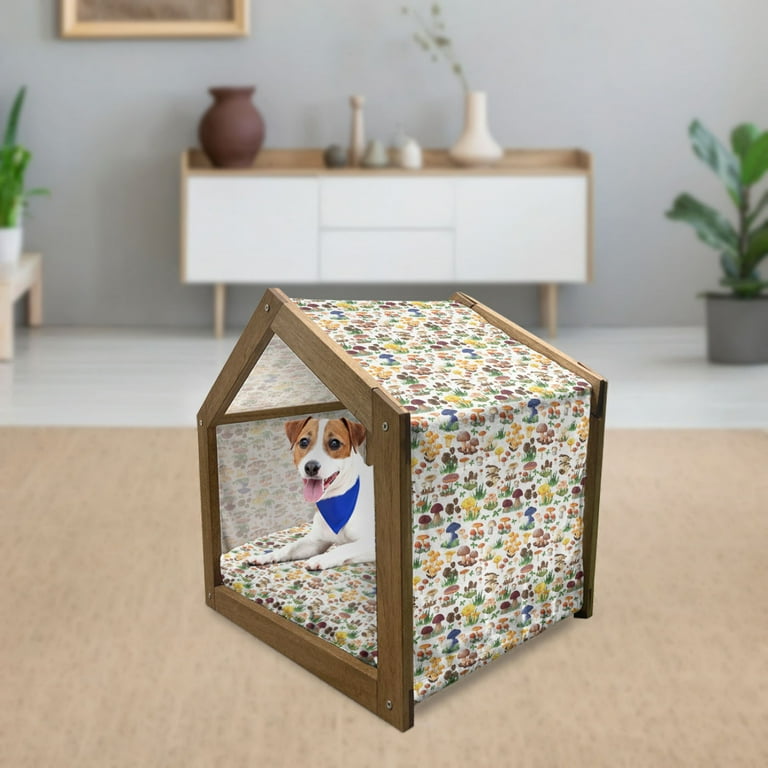The image is a square-format color photograph featuring a cozy, tent-like dog bed positioned in the center of a living room setting. The dog bed, shaped like a small house with a wooden frame, encompasses a soft cushion on the bottom and is draped with fabric adorned with a colorful mushroom pattern featuring red, blue, purple, brown, and yellow mushrooms. Inside the dog bed, a relaxed white and brown Jack Russell Terrier is comfortably lying with its paws outstretched, wearing a blue triangular handkerchief around its neck.

The dog bed rests on a light pink rug, which in turn is placed on a very light or white-tiled floor. The backdrop includes a gray wall against which stands a white and light wood wall table. On this table sits a brown vase alongside smaller white and light green vases. Flanking the table are two green plants: one in a gray pot on the floor, and the other in a white pot positioned on a piece of furniture. The scene is characterized by a blend of photographic realism and 3D illustration techniques.